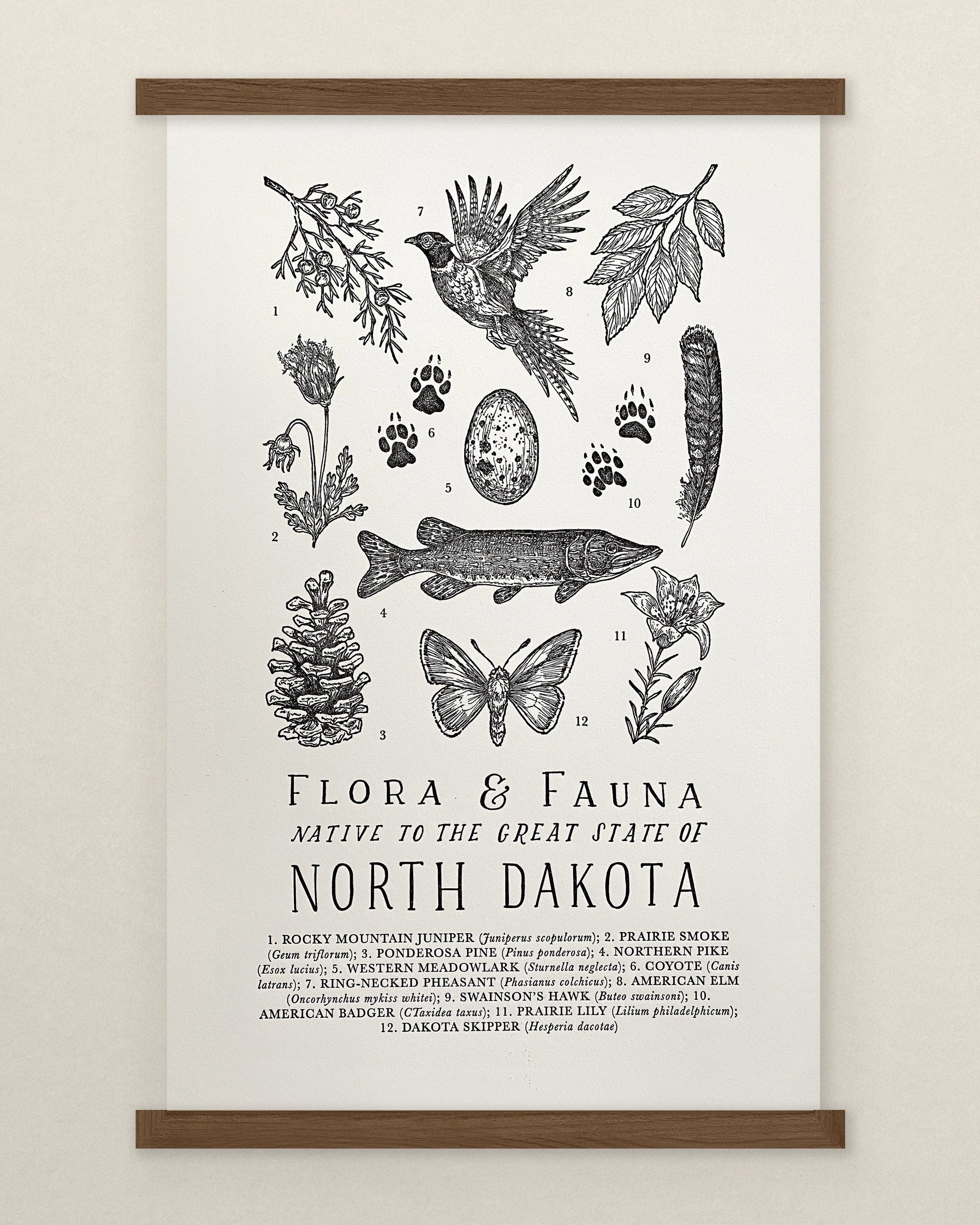A wall hanging features a meticulous black-and-white drawing set against a white background, anchored at the top and bottom by horizontal wooden supports. The artwork is composed of twelve numbered images, each with detailed depictions of flora and fauna native to North Dakota. The topmost left image portrays a twig, possibly of Rocky Mountain Juniper. To its right, a bird, identified as a Western Meadowlark, is captured in mid-flight with its wings spread wide, moving leftward. Adjacent to the bird is another leafy twig.

The bottom row begins with a withered flower, likely Prairie Smoke, followed by two sets of paw prints, potentially from a Coyote and an American Badger. Continuing along, there is a splotched egg, a distinctive feather with black and white rings, a pine cone, and a fish, possibly a Northern Pike, swimming to the right. The central images include a moth or butterfly, identified as a Dakota Skipper, lying above a pine cone (distinctly Ponderosa Pine), and a rightmost flower with small leaves, perhaps a Prairie Lily.

Below these images, the caption reads, "Flora and Fauna, Native to the Great State of North Dakota," providing a detailed description of each depicted element, including species such as the Rocky Mountain Juniper, King-necked Pheasant, American Elm, Northern Pike, Western Meadowlark, Coyote, American Badger, Prairie Smoke, Ponderosa Pine, and Dakota Skipper. This comprehensive representation celebrates the biodiversity of North Dakota, encompassing plants, animals, and insects in intricate illustrations.